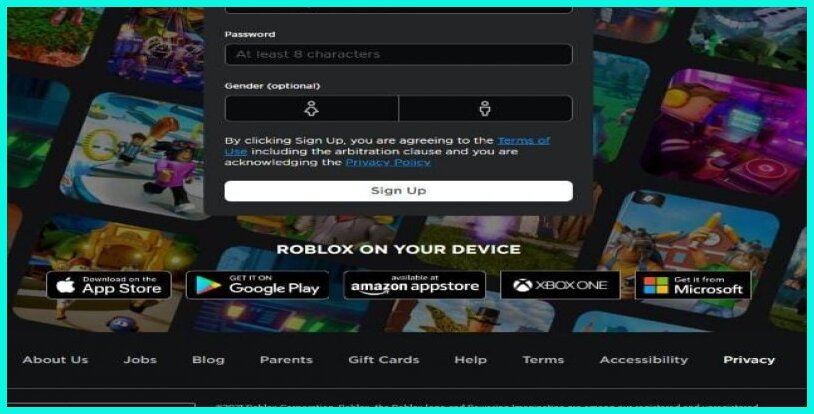The provided image showcases a webpage that appears to be for Roblox, possibly accessible via platforms like Steam or EA, though the specific source is uncertain. The background features various game images, overlaid with a cyan-blue border surrounding a central dark gray pop-up window.

The pop-up interface is intricate and contains the following elements:
- A dark gray rectangle at the top, partially cut off, leading to another prominent rectangle inscribed with the word "Password" in bold white text. This section is black with a subtle border and contains gray text indicating the requirement of at least eight characters for the password.
- Below are two side-by-side rectangles depicting gender options with silhouettes of a woman and a man. Above these rectangles is the word "Gender" in bold white text, followed by "(Optional)".
- Further down, in white text, is a disclaimer: "By clicking Sign Up, you agree to the Terms of Use (hyperlinked in blue and underlined), including the arbitration clause, and you are acknowledging the Privacy Policy (also hyperlinked in blue and underlined)."
- There is a rounded rectangular "Sign Up" button, white with black text in its center.
- At the bottom of the pop-up, "Roblox on your device" is written in bold white text.

To the left of the pop-up, a series of download options are lined up:
1. An Apple Store button featuring a white apple icon and the text "Download on the App Store" in bold white.
2. A Google Play button with a multicolored triangle icon and the text "Get on Google Play" in bold white.
3. An Amazon App Store button with the Amazon logo (from A to Z smiling face) and the text "Available on Amazon App Store" in bold white.
4. An Xbox button with a white circle and black X, labeled "Xbox One".
5. A Microsoft Store button comprising a red, blue, green, and yellow square, labeled "Get on Microsoft" in bold white text.

At the bottom of the webpage, several navigational tabs are listed, including:
- About Us
- Jobs
- Blog
- Parents
- Gift Cards
- Help
- Terms
- Accessibility
- Privacy (highlighted in bold white)

This detailed description captures the various features and layout of the landing page effectively.